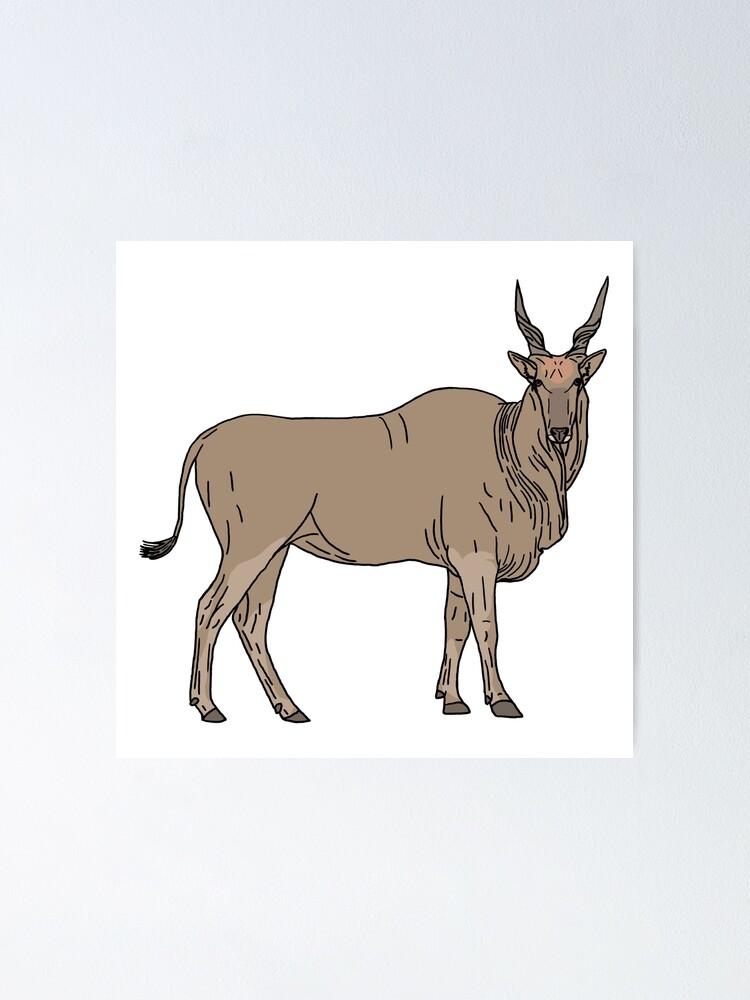The image depicts a hand-drawn, computer-generated antelope against a light grey-blue background, centered within a white square. The antelope, resembling a kudu, is shown in a detailed side view, with its head twisting to look directly at the viewer. The animal is illustrated in various shades of light brown, which blend subtly, giving it a fairly nondescript appearance. Its twisted horns, a hallmark of antelopes, rest atop a narrow head adorned with folds of skin around the neck. The antelope's body features a noticeable hump at the shoulder area and culminates in a short tail, extending halfway down its back and ending in wispy hairs. Each of its four legs, equipped with brown hooves, shows specific positioning, with the right front leg and left back leg slightly extended forward. The image does not contain any text or additional descriptive elements.